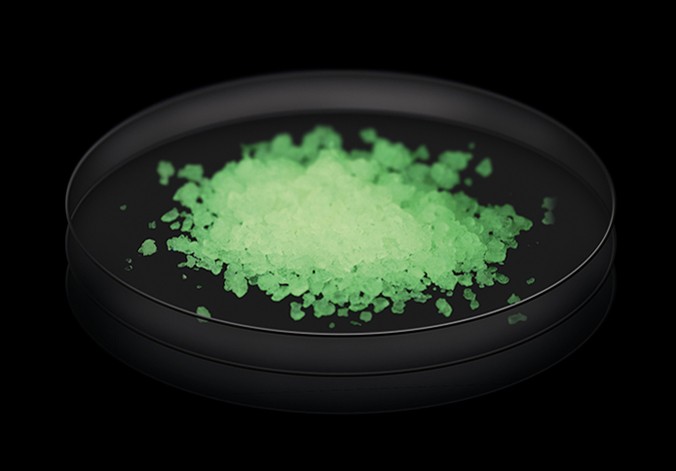The image features a circular container, resembling a saucer or the underside of a bottle cap, set against a completely black background. The main focus is a pile of crystallized material in the center of the container. The crystals appear predominantly green, though the densest part of the pile in the middle exhibits a white, glowing hue, possibly due to light reflection. Scattered around the center, the green crystals stand out starkly against both the dark container and its surrounding reflective black surface. The stark contrast and arrangement of the crystals suggest a detailed, zoomed-in view that highlights their rough and uneven texture.